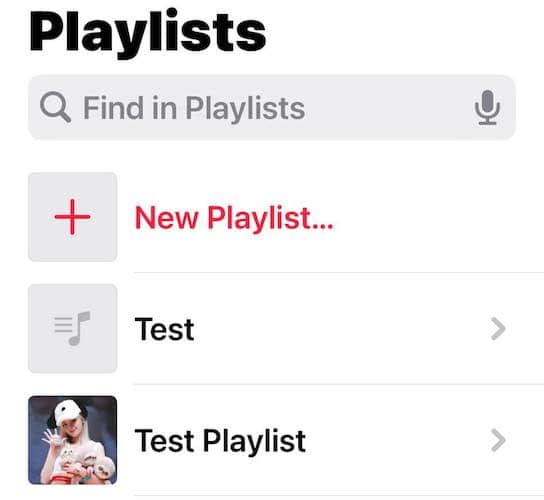At the top of the image, the word "Playlist" is prominently displayed in large, dark black letters. Below this heading, there is a horizontally extended gray rectangle featuring a search icon in the shape of a magnifying glass. Inside the rectangle, it says "Find in playlists" in gray text. To the right of this text box, there is a gray microphone icon.

Further down, there is a gray square with a red plus sign inside it. Adjacent to this square, it says "New Playlist..." in red text. A gray line separates this section from the following elements.

On the left, there is another gray square that contains a music note symbol with three lines. Next to this square, it says "Test" in black text, followed by a right arrow. Below this, another gray line acts as a divider.

At the bottom part of the image, there is a square featuring a photograph of a woman wearing a hat that resembles a panda and holding stuffed animals. The woman has blonde hair. To the right of this square, it says "Test Playlist" in black text, accompanied by a right arrow. Another gray line is situated underneath this section.

The background blends seamlessly with the interface of the website, presenting a cohesive look. The primary colors used in this image are black, gray, red, and white, with additional hints of yellow, flesh tones, light brown, pinkish color, green, and blue visible in the photograph of the woman.